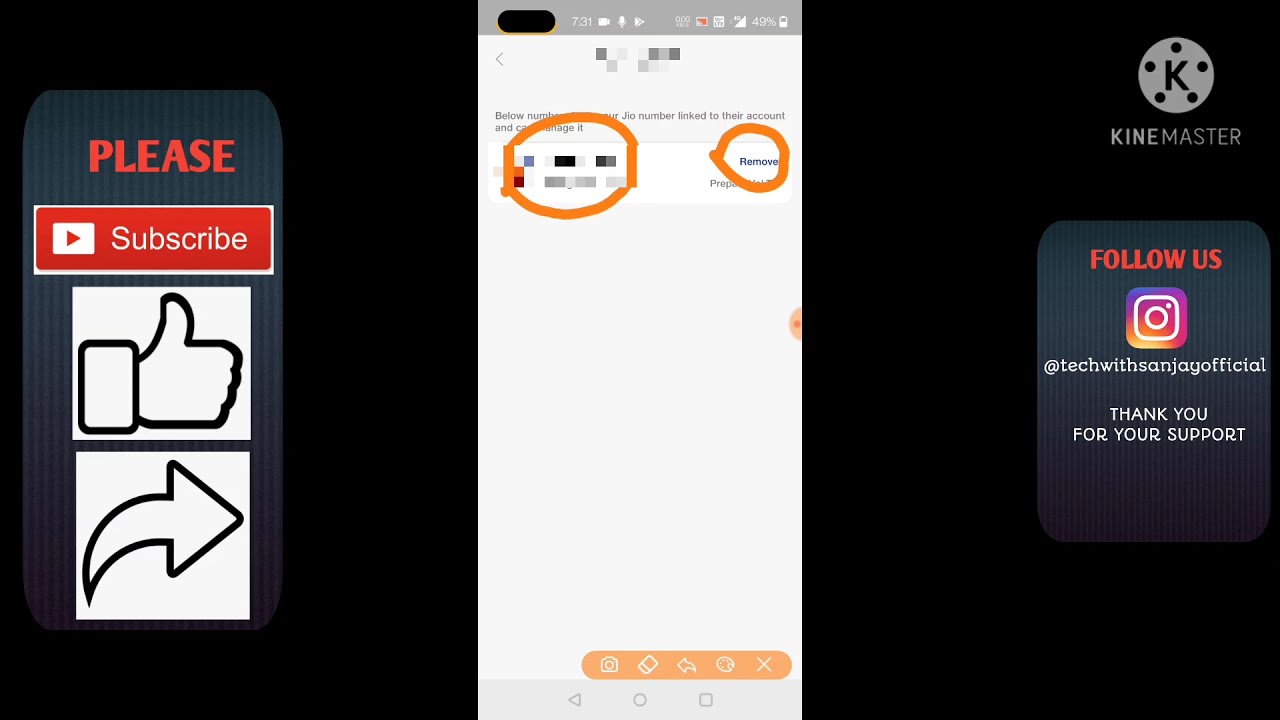The image features a central white screenshot taken in portrait mode, appearing as a screen grab from a smartphone. At the top-left corner, the display shows the time as 7:31 AM, alongside icons for a camera, a microphone, and the Google Play logo. On the top-right corner, other symbols are visible, including the signal bar, '49%', and the battery icon. Black text is faintly visible below this, partially obscured by two orange circles drawn on the screen. The bottom section of the screenshot includes a light gray navigation bar with the familiar back arrow, home button, and app switcher icons: a triangle pointing left, a circle, and a square.

To the left of this central screenshot, a vertical banner reads "please" with an arrow pointing to the YouTube subscribe button below, paired with thumbs up and share icons. 

On the right side, a "Follow us on Instagram" message is displayed, along with the Instagram handle "@techwithSanjayOfficial" and the note "Thank you for your support." Above this text is the KineMaster logo—a gray circle with a black 'K' surrounded by five black dots arranged in a star pattern—featuring "KINE MASTER" written underneath in the same gray color.